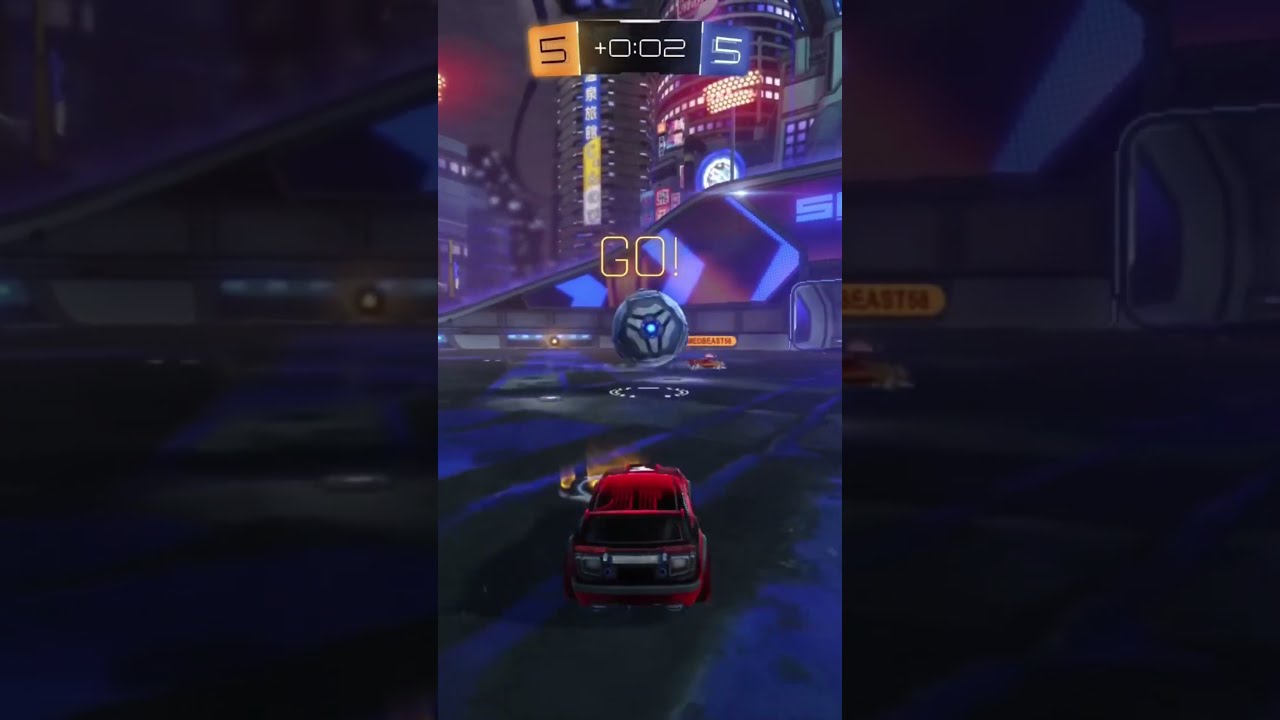The image is composed of three panels, with the center panel brightly highlighted and flanked by translucent, darkened close-ups on either side. It depicts a scene from a video game, resembling a cartoonish cityscape with vibrant neon lights. Dominating the center of the image is the word "GO!" in gold, amid a bustling city at night. A large black pavement area with dark blue streaks forms the ground. A sleek, black vehicle featuring red illuminations on the roof and red paint streaks on the sides is prominently displayed in the foreground. Above, a digital scoreboard hovers, displaying numbers and graphics: a timer at plus "0:02" and different colored squares each showing the number five. This central panel is visually clearer compared to the surrounding panels. The vehicle's rear, with detailed black and gray accents, is poised on the pavement, suggesting the start of a race, emphasizing the dynamic and competitive nature of the scene.